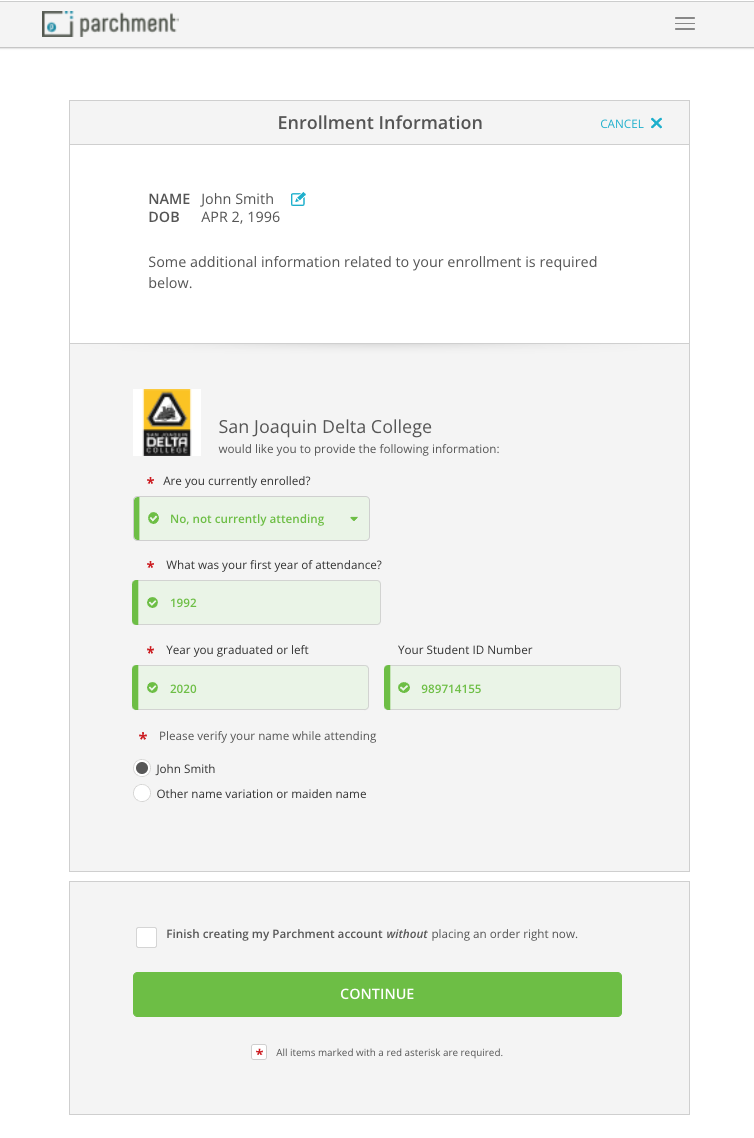This is a screenshot displaying enrollment information for San Joaquin Delta College. The header clearly states "Enrollment Information," suggesting it's an instructional example. The personal details include the name "John Smith" with a date of birth listed as April 2, 1996. The page background is a light gray, with white text fields and sections adding contrast. Highlighted responses to enrollment questions are in lime green, with one notable question being "Are you currently enrolled?" answered as "No." Towards the bottom, a large, clickable box labeled "Continue" is filled in a dark lime green shade. The college's branding is present, featuring a yellow "Delta" with a black triangle on the logo, adding a splash of color. Overall, the design remains predominantly monochromatic with strategic use of lime green and yellow for emphasis.